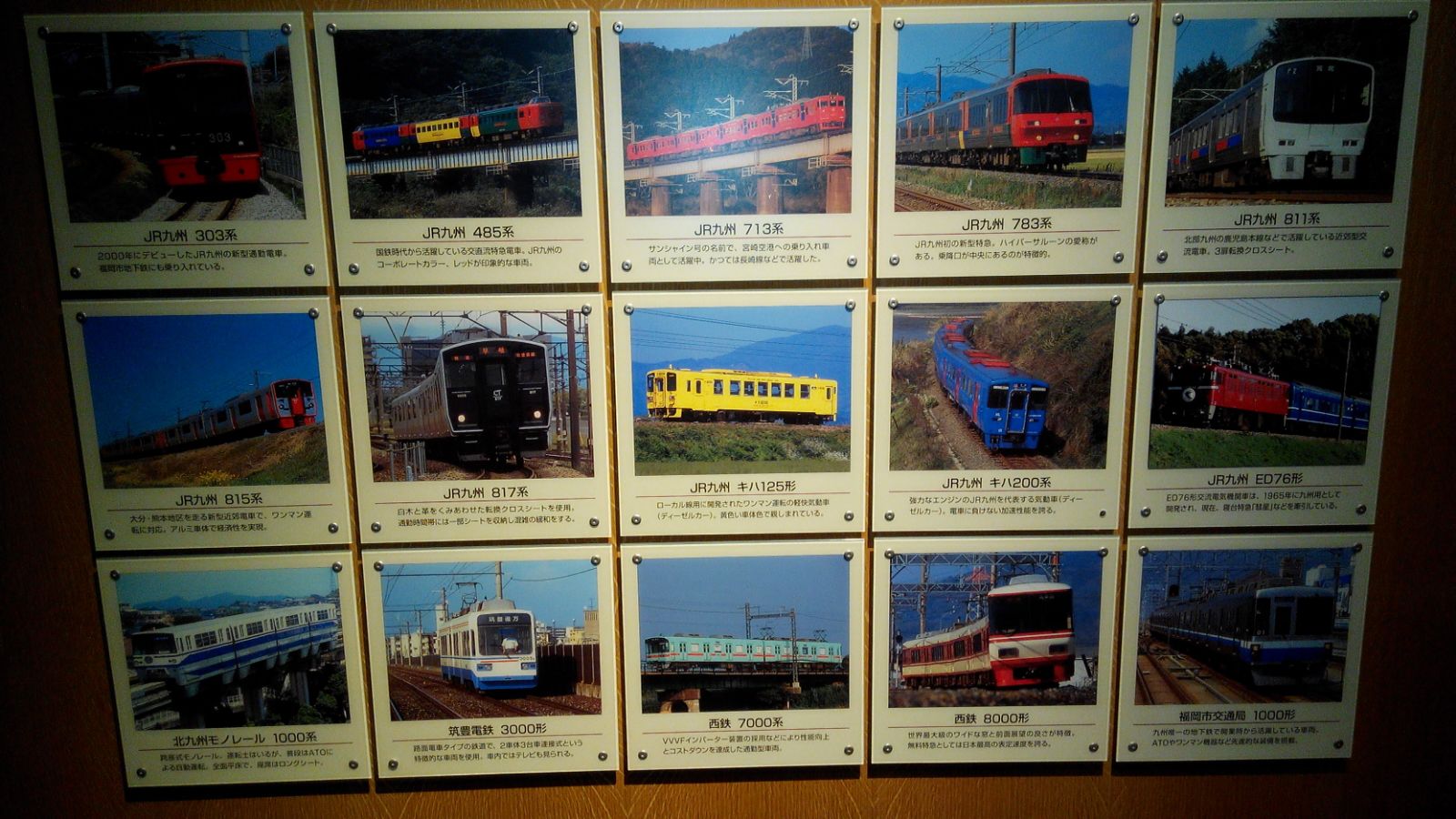This horizontally cropped color photograph showcases a brightly lit central area with darker edges, taken with a flash. It appears to display a wooden plaque, adorned with 18 metal plates, arranged in a grid of six plates across and three down. Each plate, secured by screws at the corners, features a window-pane design with a brown background. These plates house color photographs of various types of trains, including high-speed and commuter trains, each depicted in vibrant colors such as whites, reds, blues, browns, blacks, and a prominent all-yellow train. The photographs offer diverse perspectives, including front views and side views, with trains traversing different terrains like mountainous areas, over water bodies, and on elevated tracks supported by pillars. Below each image is a number accompanied by text in an Asian language, possibly Chinese. The plaque itself has an old-fashioned dark-orangey, light-brown wooden appearance, suggesting a museum or exhibition setting where enthusiasts might congregate to appreciate these train images.